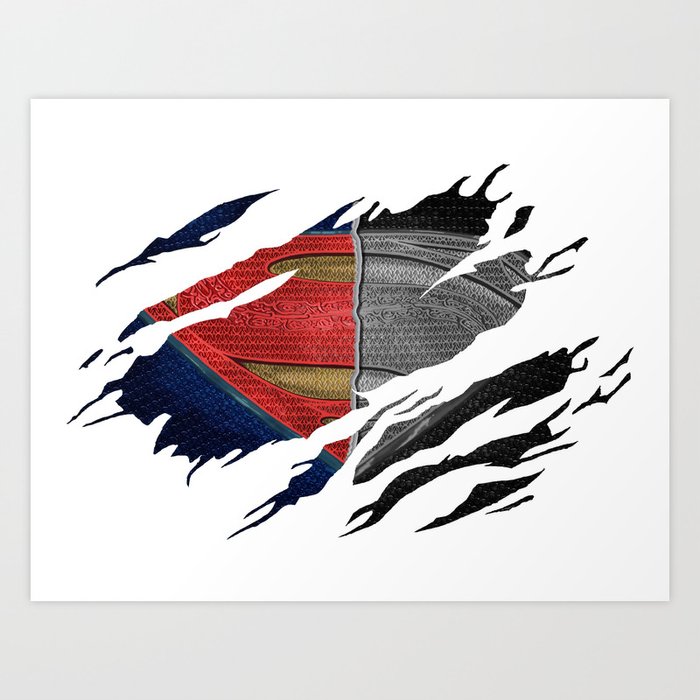This digital artwork features a close-up of the iconic Superman logo as though it is being revealed through slashed white material. The background is stark white, emphasizing the torn effect that exposes the superhero emblem. The left side of the logo is vibrant and colorful, featuring the red "S" against a yellow backdrop, all mounted on the traditional blue uniform. In contrast, the right side of the logo is depicted in grayscale, with the "S" and background rendered in medium and light gray respectively, on a dark gray uniform. The texture of the logo suggests a densely woven nylon fabric, and while the artwork gives the illusion of fabric, it has actually been drawn or digitally illustrated. The pattern within the "S" has intricate details, adding to the depth and realism of the piece.